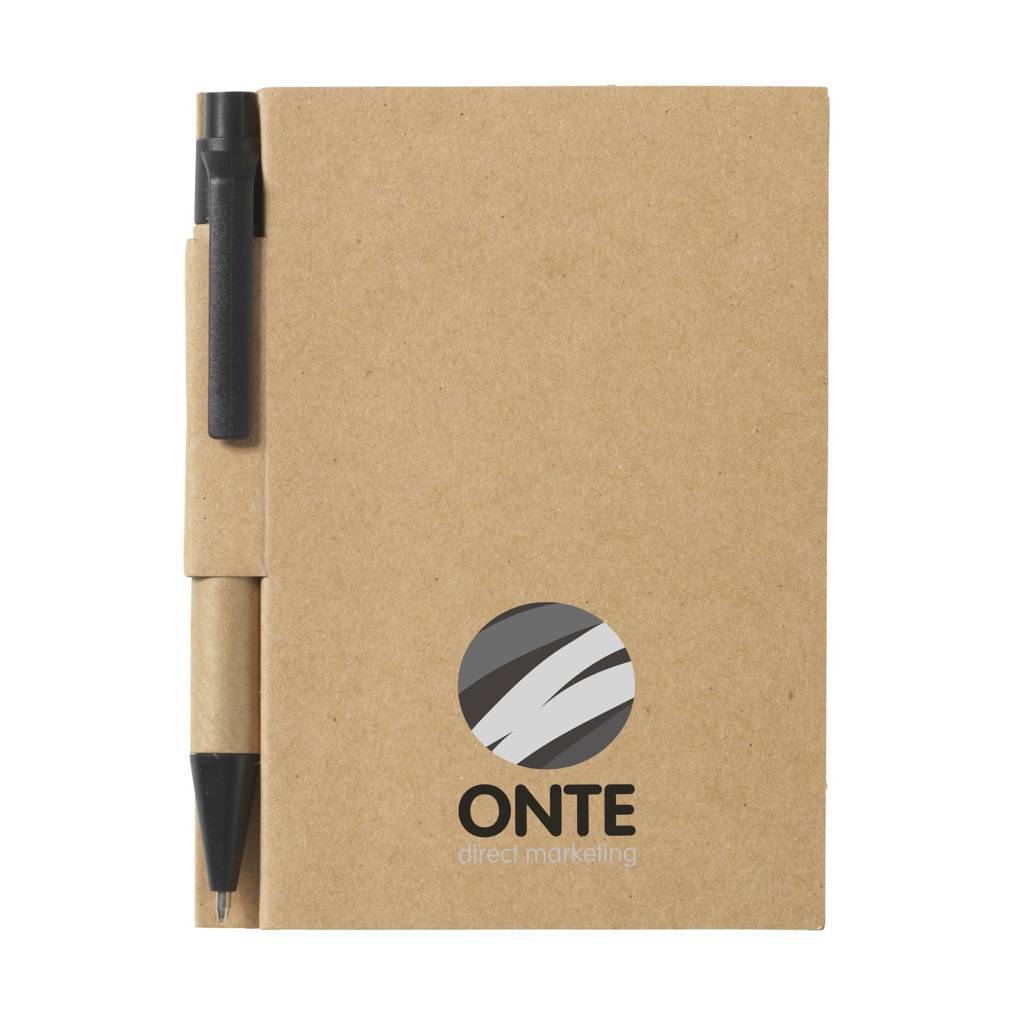This image features a simple, brown notebook resembling a recycled paper bag or cardboard. The notebook's cover is plain, adorned only with a circular logo at the bottom center. The logo comprises various lines in shades of gray and white and bears the text "O-N-T-E" in black, with "direct marketing" written underneath in white, lowercase letters. Attached to the binding on the left side is a black, click-style ballpoint pen, its tip exposed, indicating it has been clicked. The overall design suggests practicality and simplicity, emphasizing an eco-friendly, minimalist aesthetic.